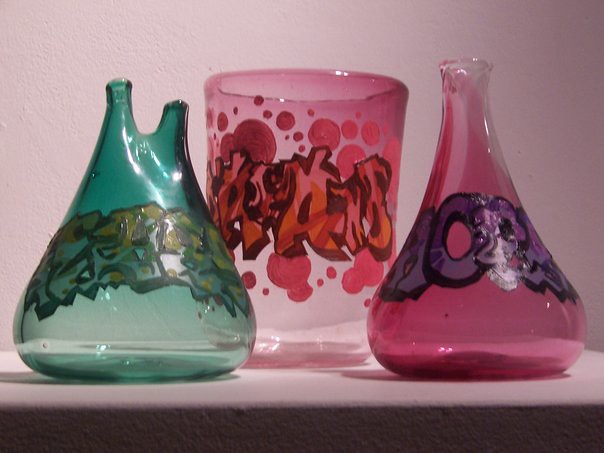The image portrays an artistic display of three uniquely designed glass vessels sitting on a light pink table against a light pink wall. Each glass features vibrant graffiti art in various colors. The left vessel is a clear teal glass with two openings at the top and yellowish-orange graffiti. Its shape resembles a beaker with a split top. The center piece is a circular, translucent pink glass with jagged graffiti in pink and red, interspersed with round reddish circles and dark outlines. The rightmost vessel is a pink, flask-like glass bottle with purple graffiti lettering stretching across its curvature. Despite their utilitarian appearances, the graffiti and design elements transform these pieces into striking art objects.